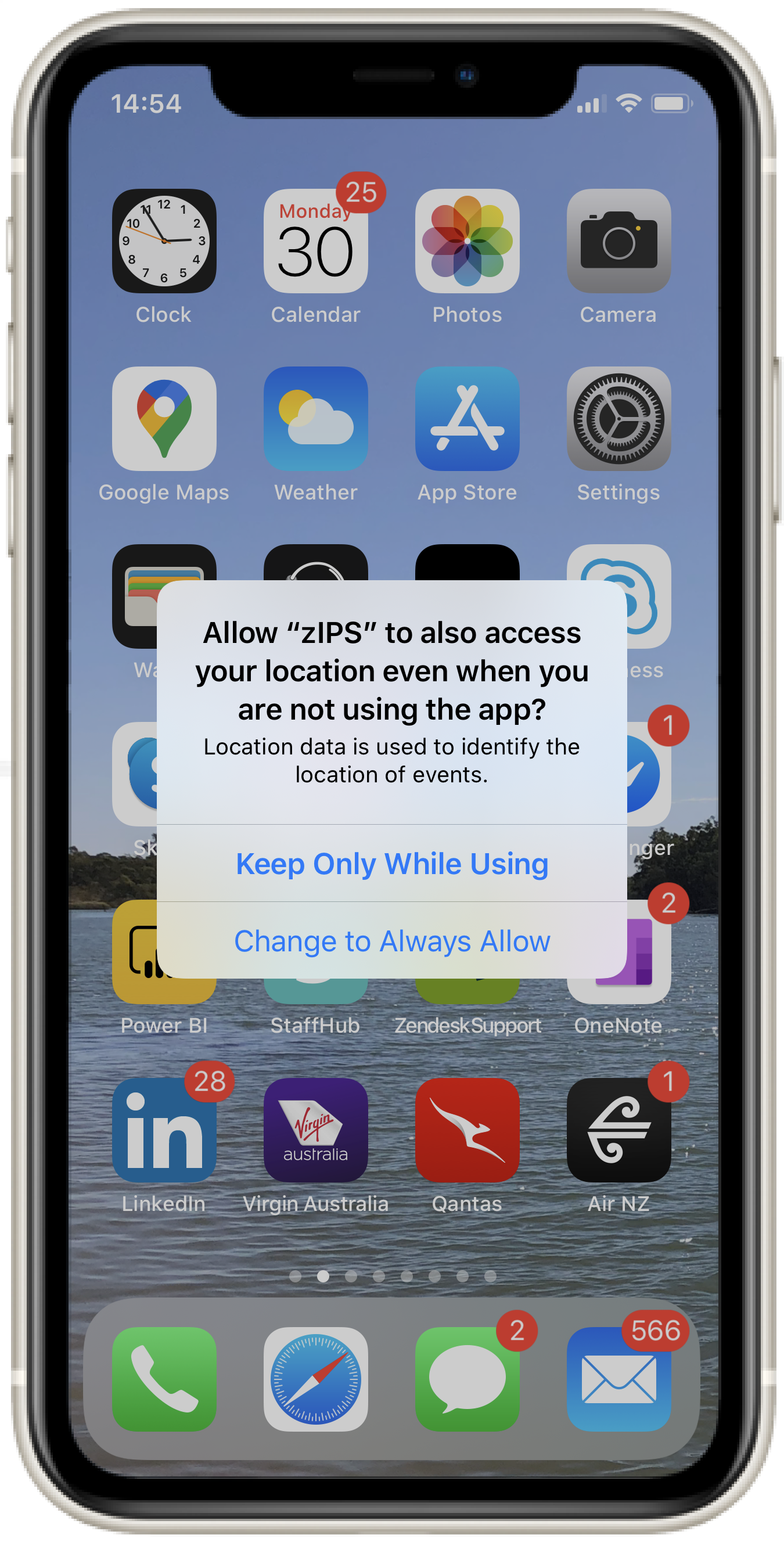In the image, we see the home screen of a cell phone with a scenic background depicting a serene body of water at the bottom, flanked by a few trees, and a light blue sky above. At the very top of the screen, the status bar shows the time as 14:54 on the left, followed by a signal strength icon with three out of four bars filled, a Wi-Fi icon in the middle, and a battery percentage icon to the right.

The home screen consists of six rows of four app icons each when viewed horizontally. The top row features the icons for Clock, Calendar, Photos, and Camera. The second row comprises Google Maps, Weather, App Store, and Settings. 

However, a pop-up dialog box in the center of the screen obscures some of the lower rows of apps. The dialog reads: "Allow Zips to also access your location even when you are not using the app. Location data is used to identify the location of events." Below this message are two options for the user to choose from: "Keep only while using" in a blue button and "Change to always allow" in another blue button.

Despite the pop-up, parts of the third row are still visible, which includes partially-covered apps. The fourth row is completely blocked by the dialog box. In the fifth row, we can see the icons for "Power Si," "Staff Hub," and two other apps that are not clearly identifiable. The sixth and bottom row shows the apps LinkedIn, Virgin Australia, Qantas, and All NZ.

At the very bottom of the screen, there is a dock with four more app icons: a Call icon on the left, followed by Safari, Messages in the middle, and an Email icon on the far right.